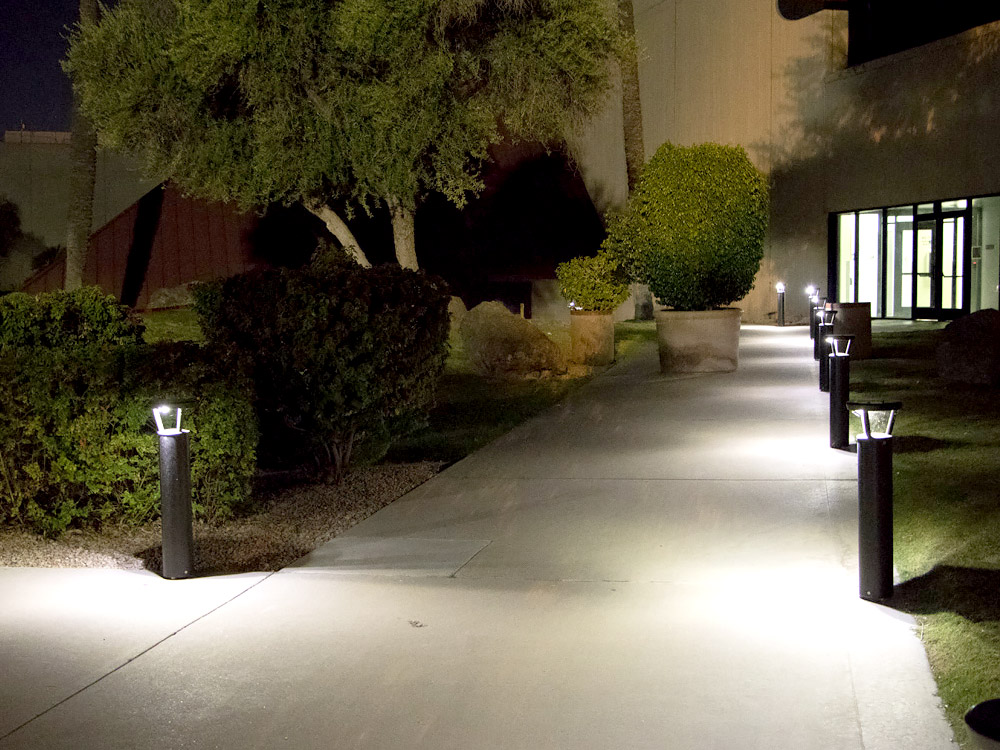The nighttime scene depicts a suburban residential area illuminated under a dark sky. In the upper left corner, a large green tree stands distinctly, accompanied by smaller green shrubs that stretch across the left side of the image. The paved ground, consisting of large white squares forming a gray sidewalk, crisscrosses through the scene. This walkway extends diagonally from the bottom of the image to the right half, making a right angle towards the left, dotted with black pillar lights that are equally spaced along the path.

On the right side of the walkway, there is a slight incline of a green lawn leading up to a building, likely a residential house, with numerous windows and glass doors emitting light. These lights, alongside the visibility of the rooftop of another house partly obscured by trees and shrubs, emphasize the nocturnal setting. A utility pole is also visible amongst the trees. The area is further illuminated by streetlights lining the sidewalk, enhancing the reflective quality of the paved ground, especially noticeable in the bottom left corner of the image.